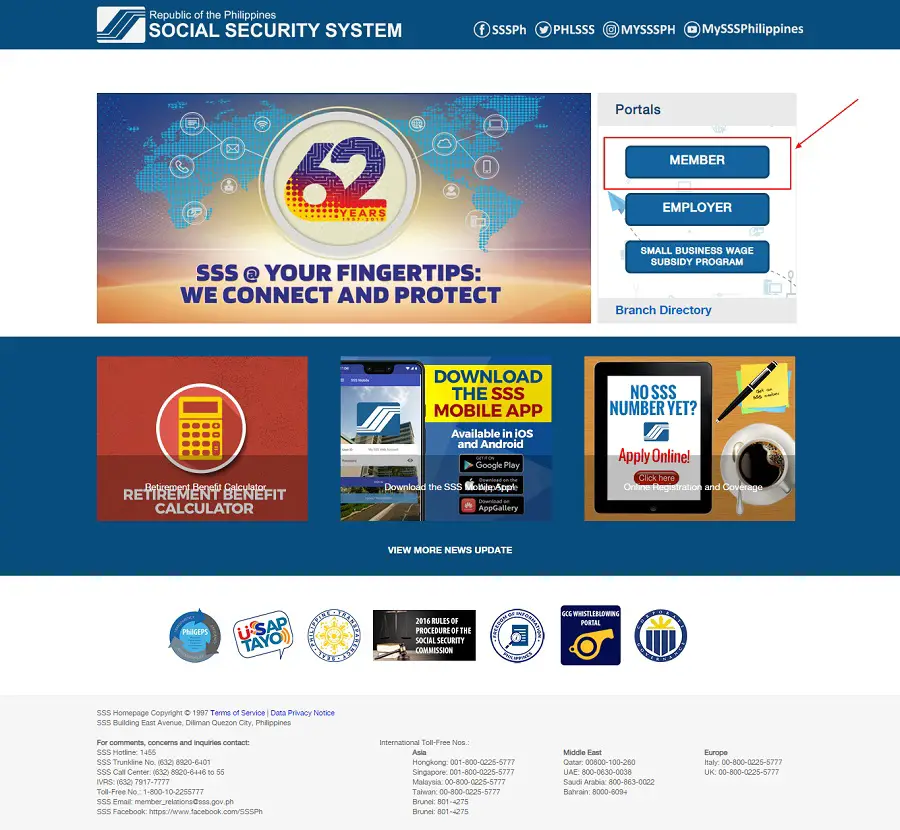Screenshot of the Social Security System (SSS) portal of the Republic of the Philippines, displayed on a white background. The portal features a blue header with "Social Security System" written in white. Below this header, there is a white square containing the SSS logo, which is a stylized "S" formed from three blue lines.

The header also includes several social media icons and handles, all in uppercase except for the lowercase 'H':
- Facebook: SSSPH
- Twitter: PHLSSS

Additionally, there is an icon labeled "ETSONMYSSSPH" and another square logo with "MySSS Philippines."

The portal layout provides various access routes such as:
- Member
- Employer
- Small Business Wage Subsidy Program

A prominent red arrow and a red rectangle highlight the "Member" section, accentuating its importance. Notably, it includes the tagline: "62 years SSS at your fingertips, we connect and protect."

Other features on this screenshot include:
- A red square with a yellow calculator icon labeled "Retirement Benefit Calculator."
- A blue square promoting the download of the "SSS Mobile App," with "Download" in blue and "SSS Mobile App" in red.

This detailed visual representation portrays the multifaceted interface of the SSS online portal aimed at providing easy navigation and accessible resources for its users.